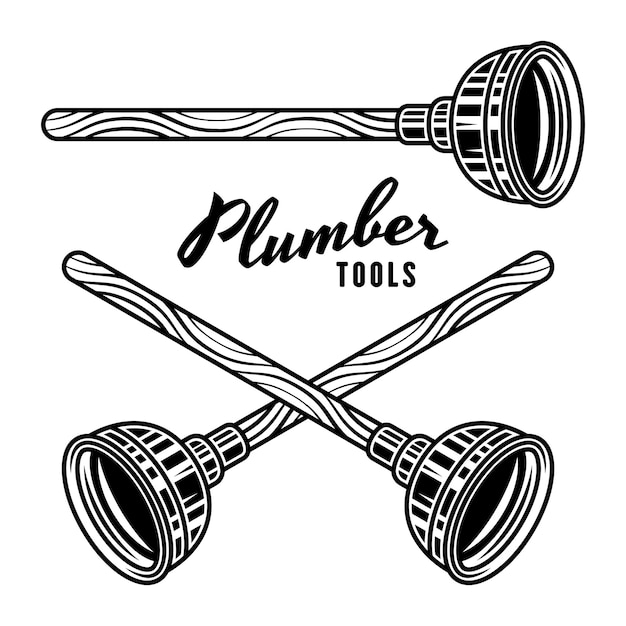This black and white graphic showcases three plungers set against a white background. At the top, the word "PLUMBER" is written in italic black cursive, while "TOOLS" appears below in all caps. Above the title, a single large plunger stands vertically, detailed with a handle outlined in black and adorned with black squiggly lines. The base of this plunger has a combination of black and white stripes, with a solid black suction cup. Below the title, two additional plungers are depicted with similar black and white striped handles and slightly darker bases. These two plungers are crossed diagonally, forming an X shape with their handles. The plungers in the image combine outlined and solid black elements, emphasizing the design's intricate use of lines to create depth and texture.